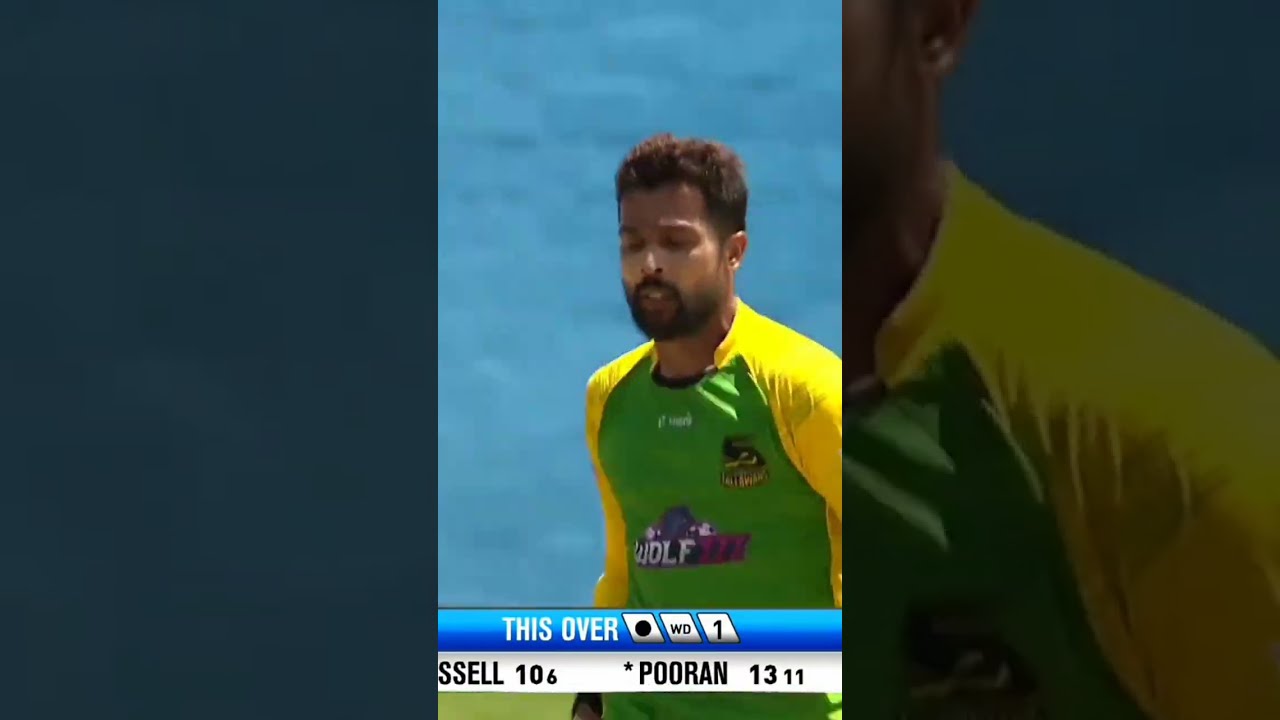This photograph captures an athlete of Indian or Middle Eastern descent, dressed in a vibrant green jersey with yellow sleeves, embellished with various logos and the word "wolf" centrally placed on the chest. The man, who has short brown hair and a short stubbled beard, is looking downward while standing on a grassy field. Behind him is a large blue background, likely part of the sports setting. At the bottom of the image, there's a scoreboard with visible text that includes "this over," "WD," and "1," followed by partially cut-off names and numbers reading "S S E L L 1 0 6," and "P O O R A N 1 3 1 1." The photo is also framed with a border made from enlarged and grayed-out elements of the image itself.